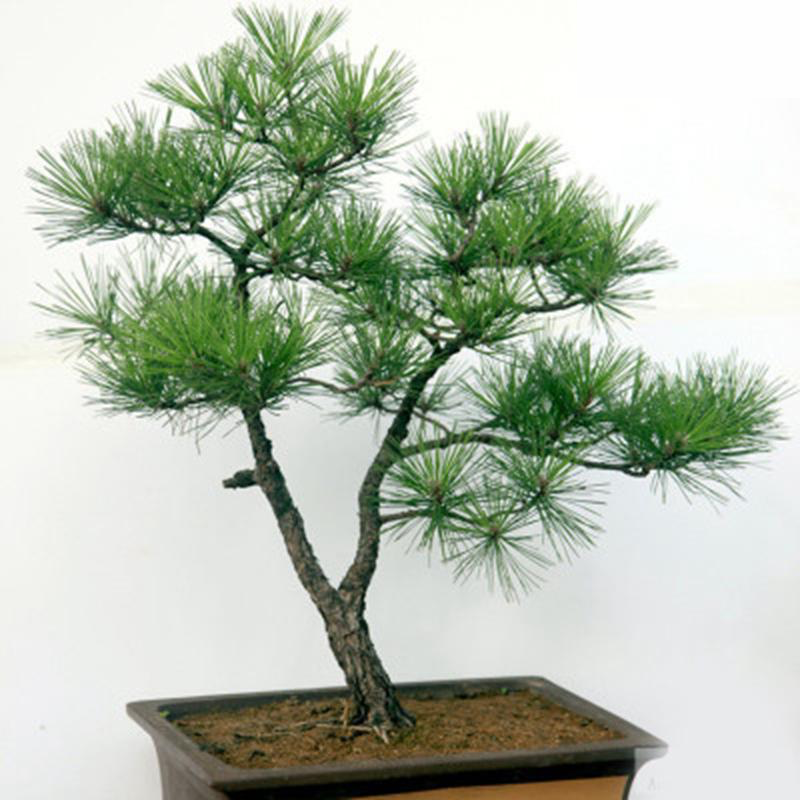The image is a close-up of a bonsai tree in a square, rectangular brown pot containing visible brown soil and small sticks at its base. The bonsai has a main trunk that splits into two primary branches, with the taller branch on the left and the shorter one on the right. Notably, the right branch features a longer, horizontal extension. Sparse, reed-like greenery is present on the branches, giving the appearance of large pine needles in contrast to the relatively small trunk. The tree leans slightly to the left, revealing its roots and brown mulch at the base. The background is off-white and out of focus, providing a simple backdrop that highlights the intricate details of the bonsai tree.